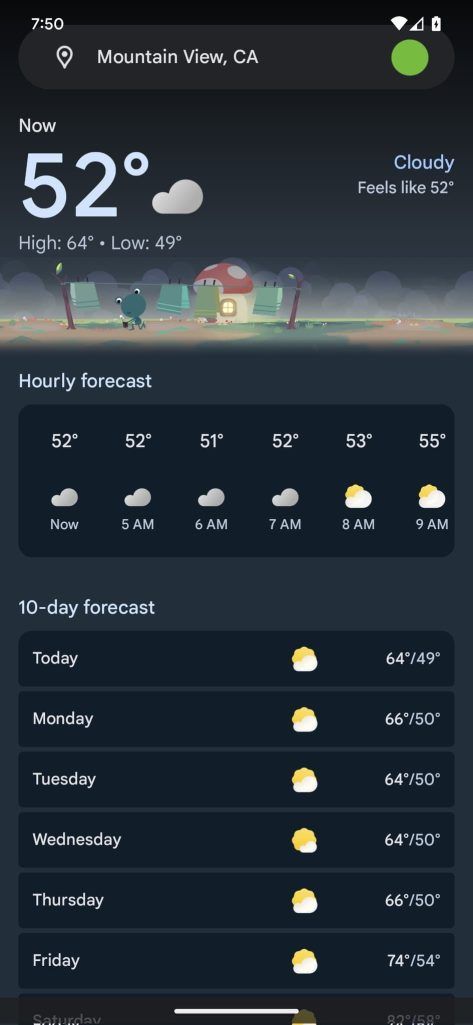Caption:

At 7:50 AM in Mountain View, California, the current weather is displayed within a search box labeled "Mountain View, California." The current temperature is 52°F with a high of 64°F and a low of 49°F. The weather is cloudy and feels like 52°F. Additionally, the hourly forecast shows temperatures ranging from 52°F to 55°F between now and 9:00 AM. The 10-day forecast predicts:

- Today: High of 64°F, Low of 49°F
- Monday: High of 66°F, Low of 50°F
- Tuesday: High of 64°F, Low of 50°F
- Wednesday: High of 64°F, Low of 50°F
- Thursday: High of 66°F, Low of 50°F
- Friday: High of 74°F, Low of 54°F

At the top of the screen are icons indicating Wi-Fi connectivity, signal strength, and battery status.